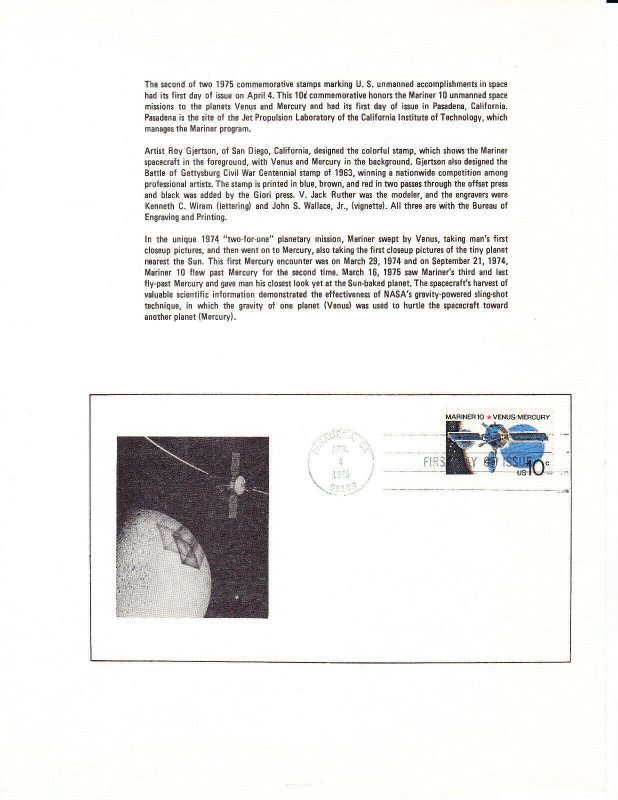This is an image of a commemorative postcard, prominently featuring a small black and white photograph of the Mariner 10 spacecraft adjacent to either the moon or a planetary body, likely representing Venus and Mercury, given the context. The postcard is postmarked in the center with the date "Pasadena, California, April 4th, 1975," and bears a 10-cent stamp designed by artist Roy Gerritsen, portraying the Mariner spacecraft in the foreground with Venus and Mercury in the background, rendered in blue, brown, and red with additional black detailing.

Above the postcard in very small letters, there is descriptive text that details the significance of the stamp, stating that it commemorates the unmanned space missions of Mariner 10 to Venus and Mercury. It highlights Pasadena as the site of the Jet Propulsion Laboratory which managed the Mariner program. The stamp, marked as the second of two 1975 commemorative stamps, honors the Mariner 10's dual planetary mission achievements, including the first close-up images of Venus and multiple encounters with Mercury, emphasizing the spacecraft's gravity-assisted trajectory.

The artistic and technical details of the stamp are also noted, mentioning that Gerritsen also designed the Battle of Gettysburg centennial stamp and that the production involved offset printing and contributions from engravers at the Bureau of Engraving and Printing. The postcard underscores the significant advancements in space exploration made possible by the Mariner missions, showcasing their landmark achievements in planetary photography and gravity-assisted navigation. The overall depiction suggests a scholarly or historical focus on NASA's space exploration history.